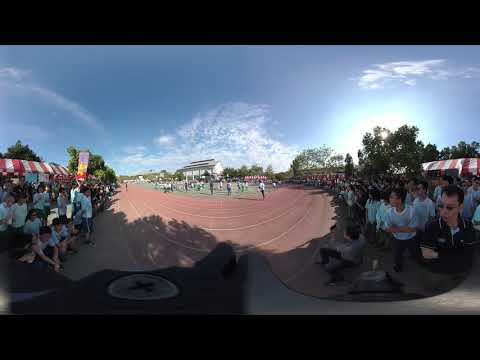The photograph showcases an outdoor track and field event, capturing a diverse crowd and vibrant surroundings. On both the left and right sides of the image, there are spectators predominantly in white or light blue shirts, many wearing black sunglasses, standing or sitting under red and white striped roof tents. The track curves through the middle of the scene, bordered by a strip of green field. The ground of the track itself is a dirt color with a hint of red. The background is framed by lush, leafy green trees with the sun subtly shining through. Above, the sky is a clear blue with a scattering of wispy white clouds. The photo is bookended by black bars at the very top and bottom, adding a distinct frame to the composition.